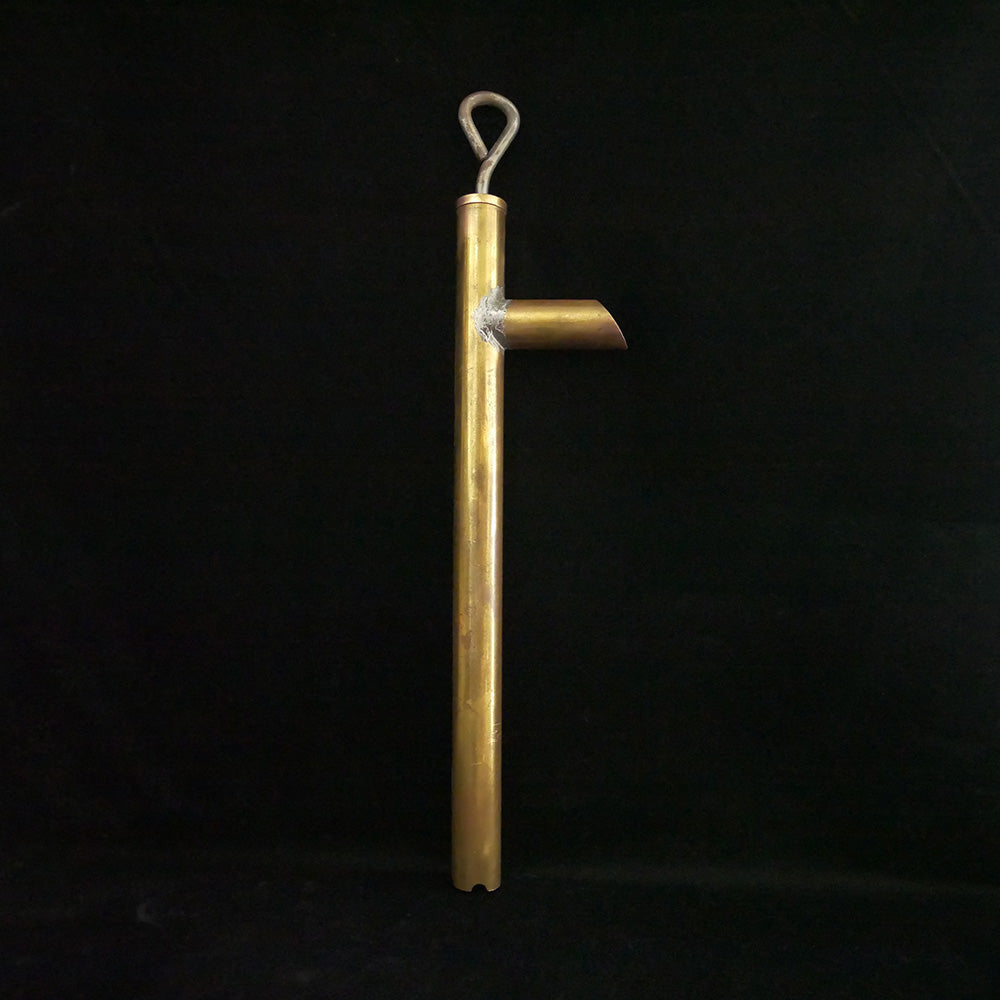The image shows a vertical copper pipe standing on a black surface with an entirely black background, giving no additional context to its surroundings. Midway up the pipe, there is a short, diagonally cut piece welded horizontally, resembling a handle. The vertical pipe culminates in a thick hook, suggesting it could be hung from a chain. The handle and the hook imply that this metallic, gold-colored pipe, resembling a tool, might be used for pushing or pulling something through the tube, similar to a caulking gun. An empty, indoor studio setting is hinted at by the descriptions but not visually confirmed.